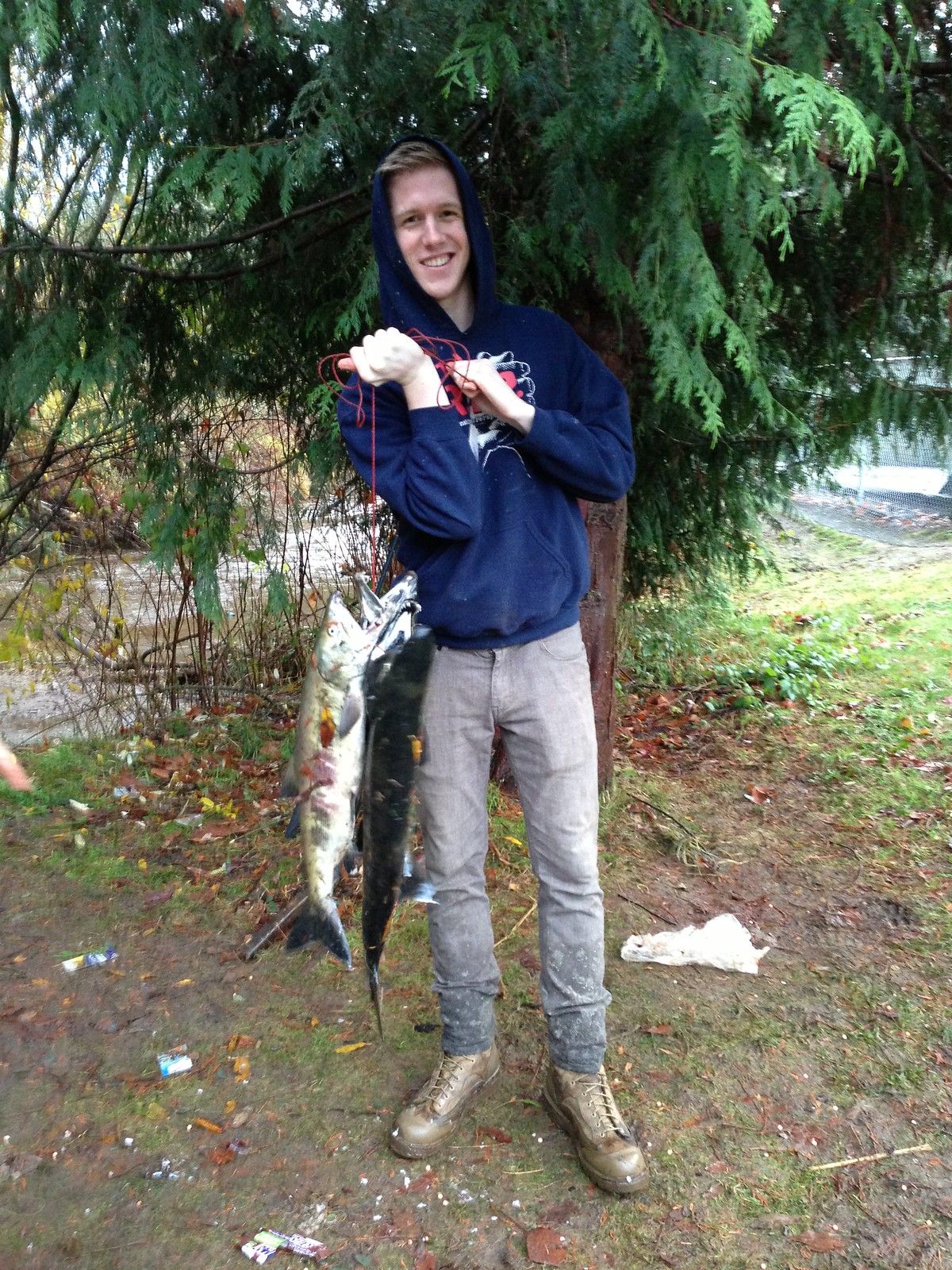In this detailed image, a young man, likely in his late teens, is posed beneath a large tree with an impressively thick trunk and long, green leaves. He stands in a grassy area scattered with bits of litter, including pieces of paper and plastic, and a body of water is visible in the background. The young man, who appears to be white, is smiling directly at the camera. He's dressed in a blue hoodie with red and white text, its hood pulled over his head, light gray jeans, and rugged, ankle-high hiking boots. Both of his hands are gripping a red string, from which three large fish, possibly largemouth bass, are suspended. These fish are nearly as long as the man's legs, indicating a trophy catch. The weight of the fish is evident as he holds them close to his chin, their heads pointing upwards and tails brushing the ground. The image captures the sense of accomplishment and the effort exerted by the young man to display his impressive catch.